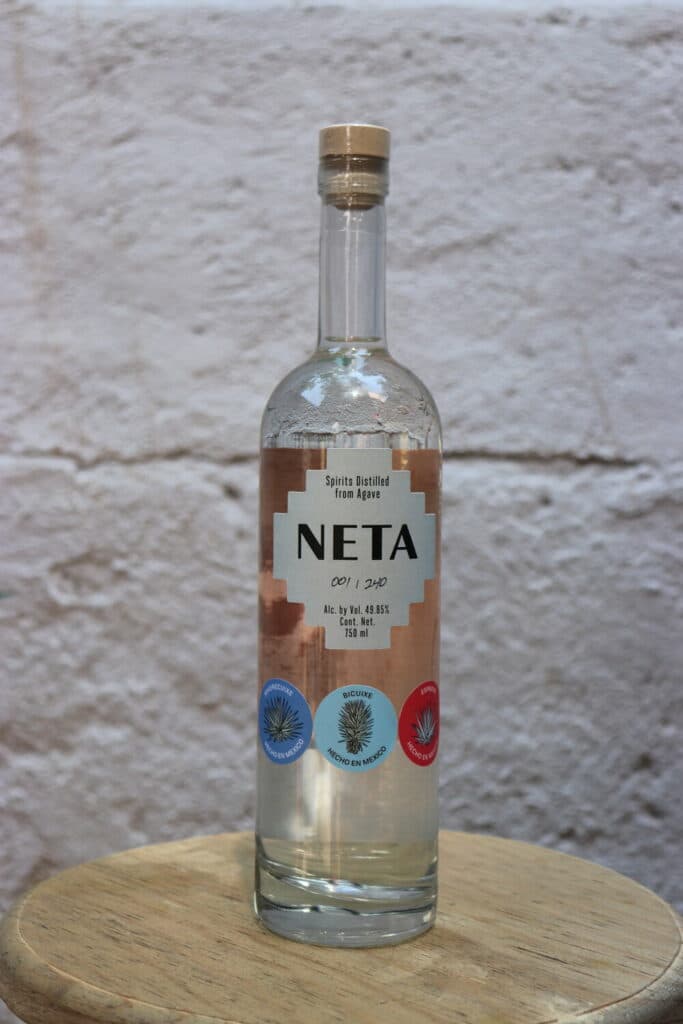This detailed image showcases a clear glass liquor bottle with a tan cork, prominently displaying a copper-colored label. The label features the brand name "META" in bold, black font, with the words "Spirits Distilled from Agave" beneath it. The alcohol by volume is marked at 49%, with a limited edition number "001 out of 240" inscribed on the bottle. At the bottom part of the bottle, there are three circular stickers, each depicting an agave plant, in blue, light blue, and red colors respectively. The bottle is filled with a clear liquid and is placed upright on a small wooden round table against a white brick wall, suggesting a rustic yet clean setting, possibly indoors.